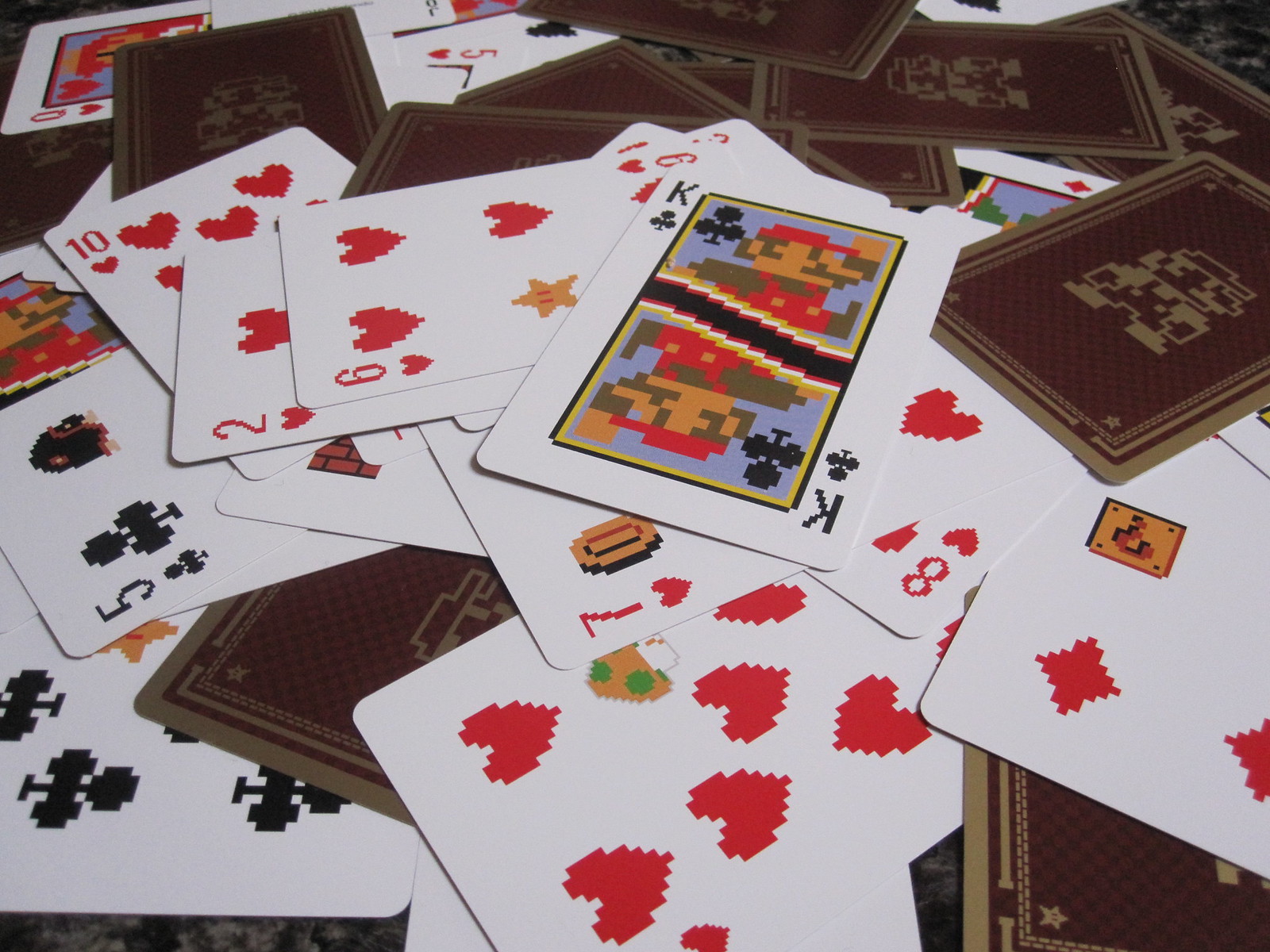This image showcases a unique deck of playing cards, evidently custom-made and possibly printed at home. The cards maintain the conventional size of standard playing cards, but diverge from traditional designs by incorporating characters from the Super Mario Bros. series. The face cards feature distinctive Super Mario-themed illustrations; for instance, the King of Clubs is represented by Mario himself, donning his iconic red hat and suspenders, depicted in a dynamic, jumping pose mirrored at both the top and bottom of the card.

The backs of the cards are brown and adorned with the image of a Koopa, one of the recognizably classic adversaries from the Mario series. Uniquely themed suit symbols replace standard symbols; for example, a card typically featuring multiple diamonds instead showcases a single iconic question mark block from the game. Another card displays a Koopa shell in place of its traditional symbols. This deck is a creative fusion of the cherished Mario Bros. universe and the format of a traditional playing card deck, resulting in a playful and nostalgic homage to the beloved video game series.